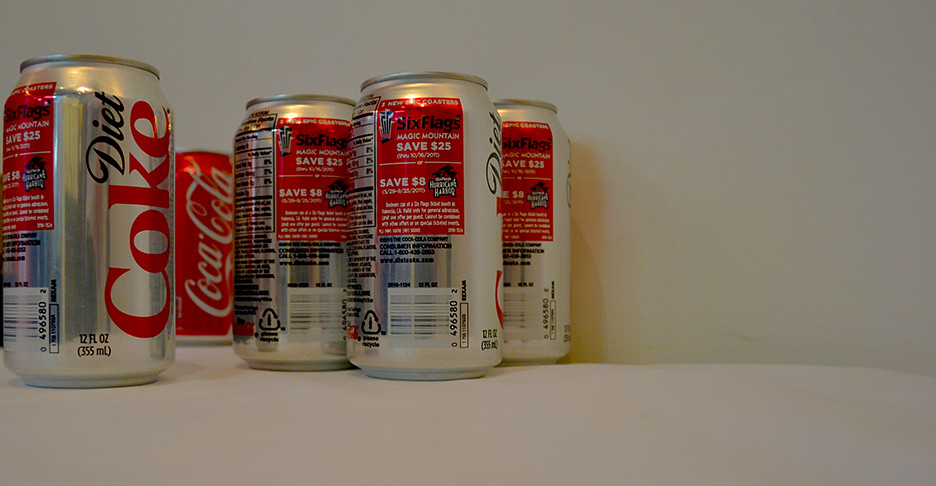The photograph captures a group of soda cans resting on a white surface against a white wall. The arrangement includes prominently featured Diet Coke cans and a single full-sugar Coke can in the background. The Diet Coke cans are silver with the word "Diet" printed in black font, and "Coke" written in bold red letters. The cans also display a detailed advertisement in red, black, and white fonts promoting a $25 saving offer at Six Flags Magic Mountain. The silver cans cast visible shadows on the wall, highlighting the overhead glare presumably from an artificial light source. In the background, a distinct red can with white lettering identifies itself as a full-sugar Coke. Each can is a standard 12-ounce size, and the nutrition labels on the Diet Coke cans use black text on a silver background. The overall scene is illuminated brightly, showcasing the intricate details and clear shadows of the cans.